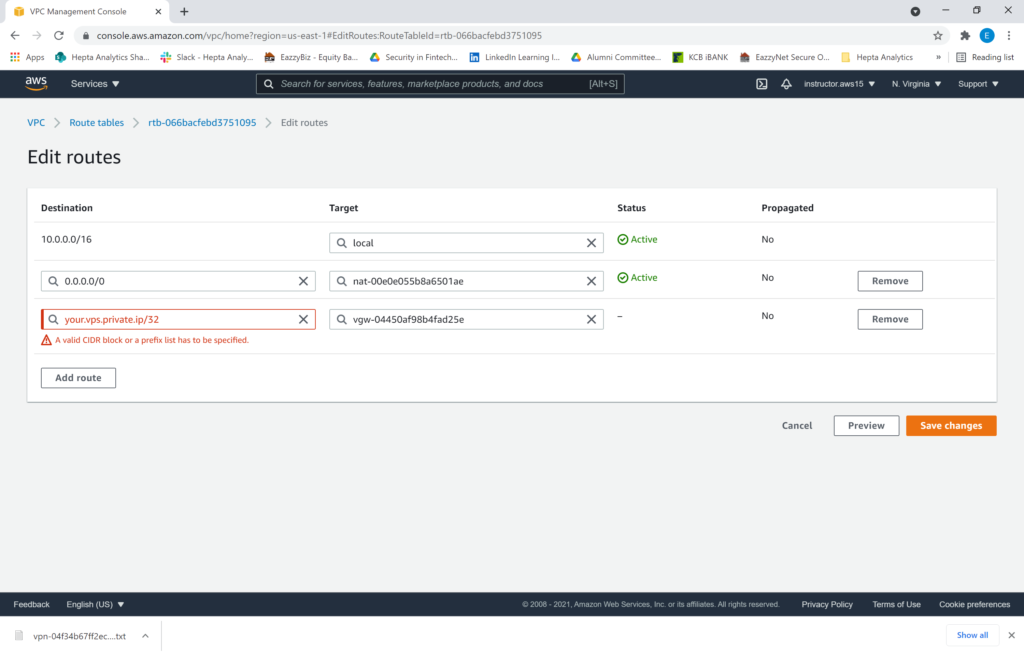A detailed screenshot of the AWS Management Console specifically within the VPC Management section. The website URL displayed is "console.aws.amazon.com," with additional paths and parameters following in gray text. The page focuses on VPC route tables, highlighting "rtb-" followed by an alphanumeric string representing the route table ID. The section of the console for editing routes is visible.

In this editing section, there are multiple routes listed with their respective details:
1. The first route has the destination set to "10.0.0.0/16," targeting "local." The status of this route is marked as "active," and it is not propagated (indicated by "No").
2. The second route has the destination "0.0.0.0/0," targeting "NAT-" followed by another alphanumeric string. This route is also marked as "active" in status but is not propagated.

Beside each route entry, there's a "Remove" button enclosed in a rectangle, allowing for the deletion of the specific route. The list continues with more items that similarly detail their respective destination subnets, targets, statuses, and propagation settings.